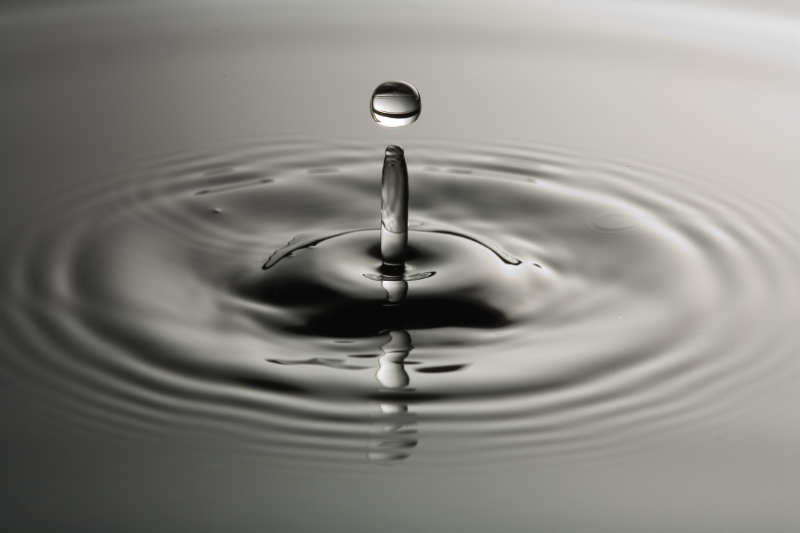In this striking black and white photograph, which is rectangular and oriented horizontally, we are presented with an extreme close-up view of a single water droplet impacting a flat water surface. The droplet is captured in midair, perfectly spherical, just before merging with the body of water below. At the center of the image, concentric rings ripple outward from the point of impact, illustrating the motion and energy of the droplet's descent. Three distinct rings are visible, adding a dynamic sense of movement to the still image. A reflection in the lower central part of the photograph mirrors the falling droplet, enhancing the scene's symmetry and depth. The composition's lighting varies, with the lower left and upper left corners veiled in darker shades of gray, while the upper right corner gradually lightens, adding contrast and visual interest to the monochromatic palette.